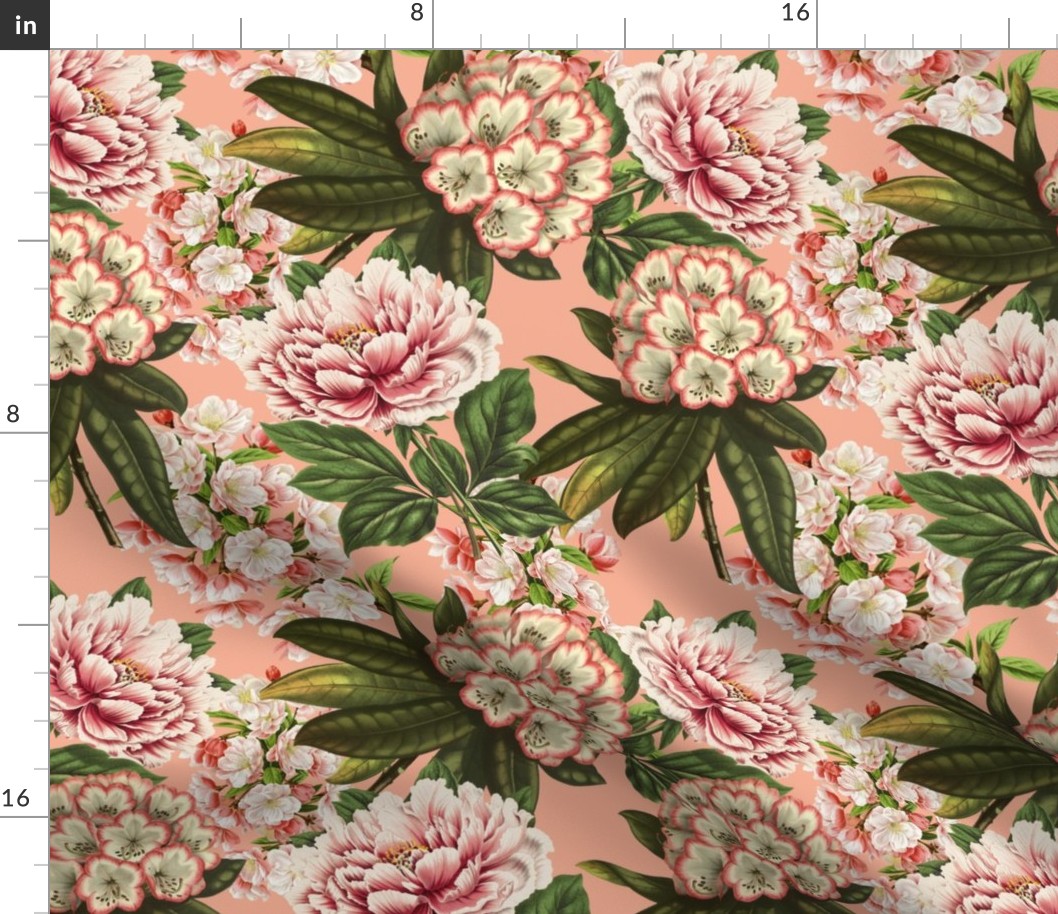The image showcases a floral printed fabric with detailed measurement notations and a vibrant array of flower designs. At the top of the picture, marked in a black box with white text, are notations indicating inches. These include sequential hash marks with key numbers such as 8 and 16 on both the left and right sides. The fabric's background is a soft peach or light pink color, setting a delicate canvas for the floral motifs.

The flowers are prominently white and pink, with some exhibiting thick petals and vibrant pink centers highlighted by small yellow buds. Interspersed among these are smaller flowers with white petals edged in pink. The green leaves present vary in shape and size, some being long and pointy while others are attached to flower stems, adding to the lush appearance. The picture captures a balance of blooms and foliage, with green leaves emanating from various points – center, upper right, lower right – intertwining through the composition and creating a dynamic interplay of color and form.